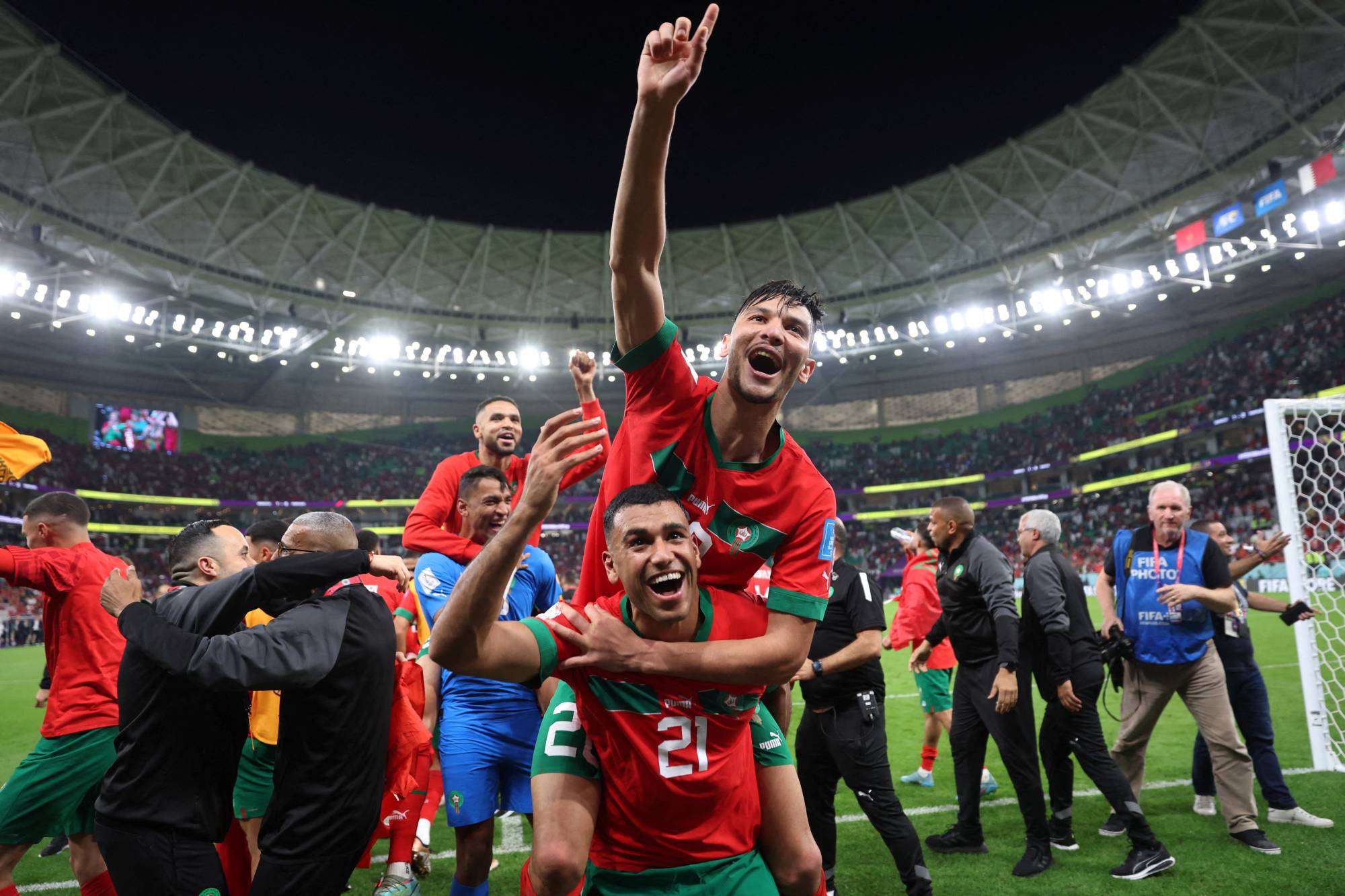In this vibrant color photograph, a joyous celebration unfolds after a soccer match in an open dome stadium under a dark night sky. The foreground features two ecstatic soccer players. One player, sporting a short-sleeved red jersey with green accents and the number 21 emblazoned on the chest, stands with a broad smile and raises his right hand triumphantly. Climbing on his back is another jubilant player, also in a red and green jersey, pointing his index finger skyward and wrapping his left arm around his teammate's chest. Both exude sheer happiness. Surrounding them, numerous people in black tracksuits, perhaps coaches or staff, hug and rejoice. The background reveals a stadium teeming with spectators and illuminated grandstands. A white-painted goalpost is visible on the right, and patches of green grass add to the scene's vividness. Among the crowd, a man in a blue vest, possibly an umpire or coach, and other players in red and green uniforms contribute to the contagious celebration, while one elderly man stands apart, staring into the distance.